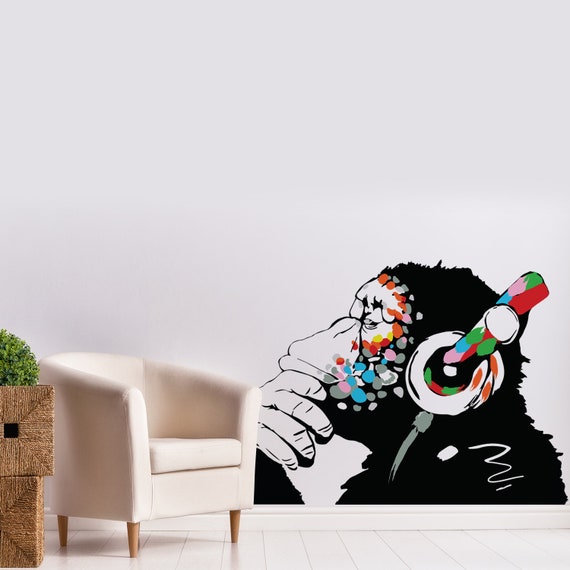This color photograph captures an artistic scene set in a stark, minimalist interior room. The background features a pristine white wall adorned with a detailed side profile painting of a chimpanzee. The chimp is depicted in a relaxed pose, with its right hand thoughtfully resting on its chin and its eyes closed, as if immersed in the music from the over-the-ear headphones it wears. The headphones are vibrant, decorated with splashes of green, blue, pink, orange, and red.

The floor, a white tile that extends seamlessly from the wall, is interrupted on the left side by a cream-colored armchair with small wooden legs, suggestive of a leather texture. Adjacent to the armchair, closer to the left edge of the image, are two stacked, woven burlap boxes, the top one topped with a lush green plant. Along the edge of the wall runs a white baseboard, completing the clean, monochromatic look of the space, which is dominated by the whimsical yet serene chimpanzee mural on the right side.